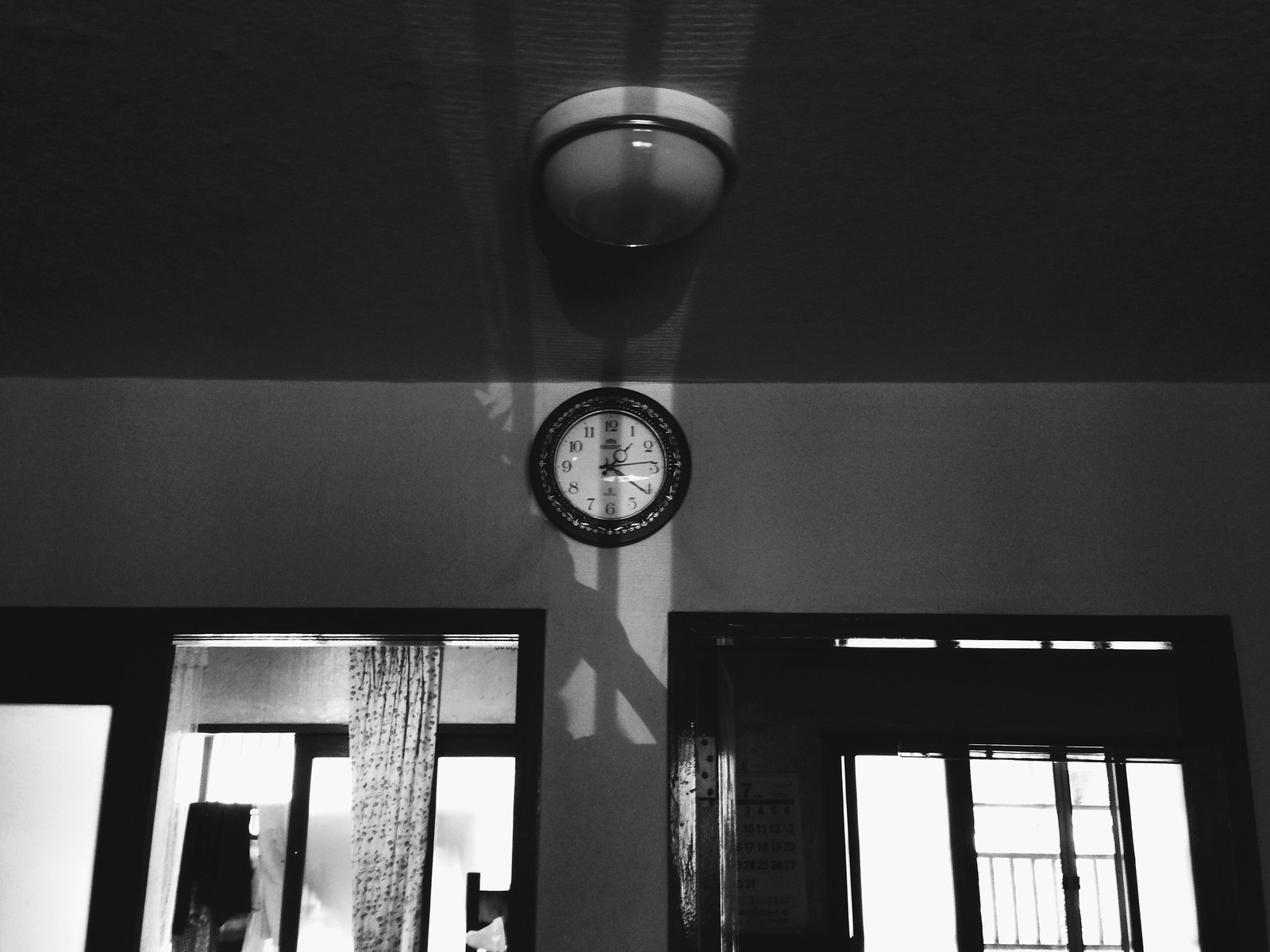This black and white photograph captures an indoor scene illuminated by sunlight streaming through two large windows, one to the left and one to the right. The light creates a reflection on the wall, enhancing the central focus of the image: a black-ringed clock with a white face, mounted prominently in the center of the wall. The clock, featuring numerical markings from 1 to 12, indicates the time as approximately 1:21. It has a distinctive design with a wide black border, a fancy hour hand that includes a needle end and a circular opening near its tip, a longer black minute hand, and a red second hand. The wall behind the clock is bathed in light, making the clock stand out against the grey ceiling and the contrast of the black and white walls. There is a simple dome light on the ceiling, which is turned off. Below the clock, a long, floral patterned curtain in black and white hangs next to one of the windows but does not obscure the light from the glass panes behind it. Against a pole near the clock, there appears to be some form of writing or a sign, though the letters are indistinct.